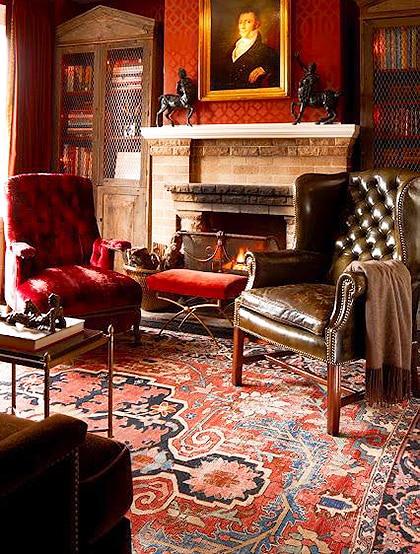This indoor photograph captures a cozy, opulent room, likely part of a mansion or large home, centered around a prominent, active stone fireplace with a white mantle. Above the fireplace hangs a golden-framed portrait of a man, flanked by two statues of centaurs, contributing to the grand atmosphere. The mantle is further adorned with shiny brown statues, appearing to be representations of horses or persons on horses. The room features an intricate, mostly red, blue, and white patterned rug, reminiscent of an Aztec or Persian design, extending before the fireplace. 

Arrayed around the rug are elegant furnishings, including a small red velvet stool or table placed centrally, a matching red velvet chair to the left, and a shiny brown leather chair to the right. Another sofa chair is situated in the bottom right corner. Flanking the fireplace are enclosed bookshelves with visible books behind metal grates, adding a vintage touch. A brown coffee table with a statue of a reclining figure atop a book rests to the left, near the chairs. The overall setting exudes an antique, stately ambiance, highlighted by the warm, inviting fire, and dark, ornate decor.